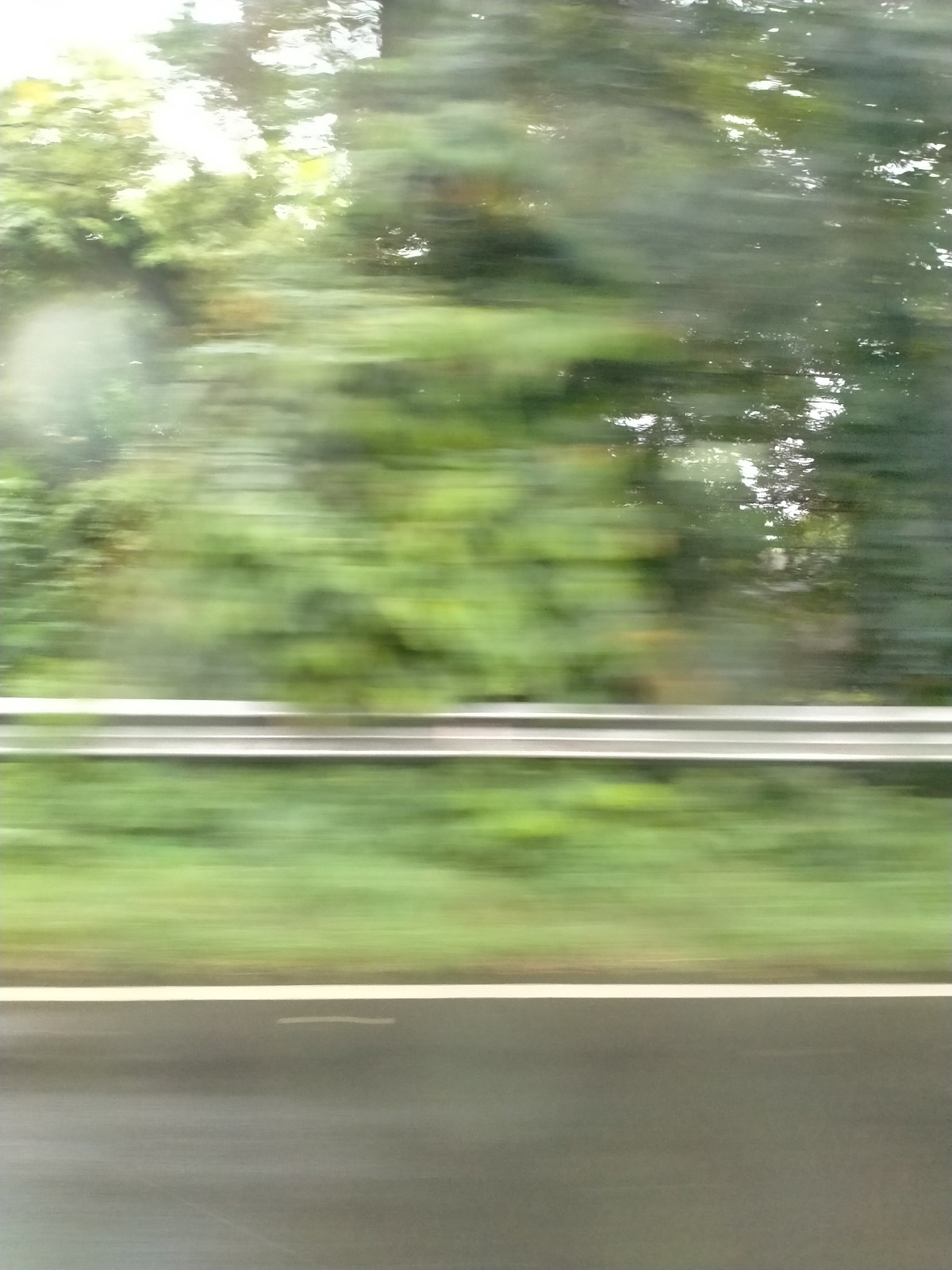This blurred photograph likely taken from a moving car captures a partial view of a sunlit road flanked by a gray metal guardrail and a white edge line. The tarmac can be seen in the foreground alongside a stretch of overgrown green grass, which leads up to thick, green tree foliage. The foliage, in various shades of green and hints of yellow, is illuminated by daylight that creates spots of light and a lens flare effect, particularly in the right corner of the image where the sunlight washes out the sky. The overall motion blur suggests the photo was taken while the camera was in motion, contributing to the soft, streaked appearance of the trees extending to the left and the scattered pockets of sunlight shimmering through the dense leaves. The scene is devoid of cars or other objects, focusing solely on the blending hues of the natural landscape and the structure of the road.